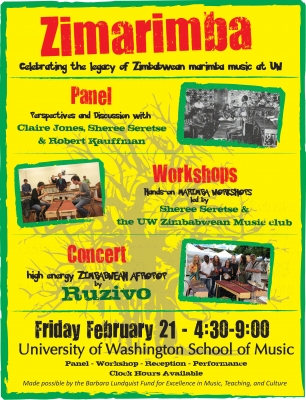The poster has a vibrant yellow background framed with a green border, showcasing red and black text throughout. At the top, bold red text announces "Zamarimba." Directly below, black text reads "Celebrating the Legacy of Zimbabwean Marimba Music at UN." Structured into sections separated by green lines, the first section titled "Panel" lists a "Perspective and Discussion with Charlie Jones, Sherry Serente, and Robert Kaufman." The next section, "Workshops," is followed by "Concert High Energy Zimbabwean Afro by Bruzevo." Towards the bottom, the poster details the event schedule: "Friday, February 21st, 4:30 PM to 9 PM, University of Washington School of Music," highlighting panel discussions, workshops, receptions, and performances. A subtle gray tree design decorates the background.